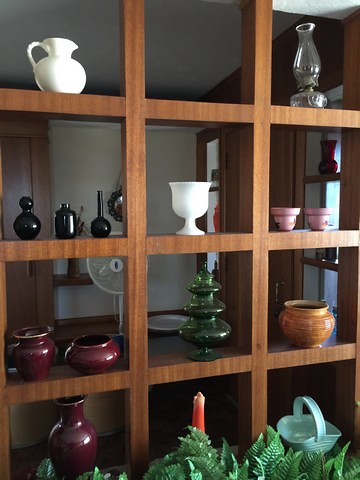This color photo features a light brown wooden bookshelf designed like a tic-tac-toe grid with three columns and four rows, housing a variety of knick-knacks within its 12 square compartments. Starting at the top left, there's a small white ceramic jug with a handle. The middle top compartment is empty, and the top right holds an old clear oil lantern with a circular base. On the second row, the left compartment contains three small black vases of varying shapes and sizes. The middle compartment houses a white glass chalice-like cup, while the right compartment holds two pink ceramic cups.

Moving to the third row, the left compartment has two maroon vases: one narrow and the other round. The middle compartment contains a green glass ornament resembling a Christmas tree. The right compartment has a short brownish-gold vase. The bottom row starts with a round maroon flower vase. The middle compartment features a single orange candle, and the rightmost compartment has a bluish ceramic basket with a handle. Surrounding the base of the bookshelf, you can see green leafy plants, adding a touch of nature to the scene.